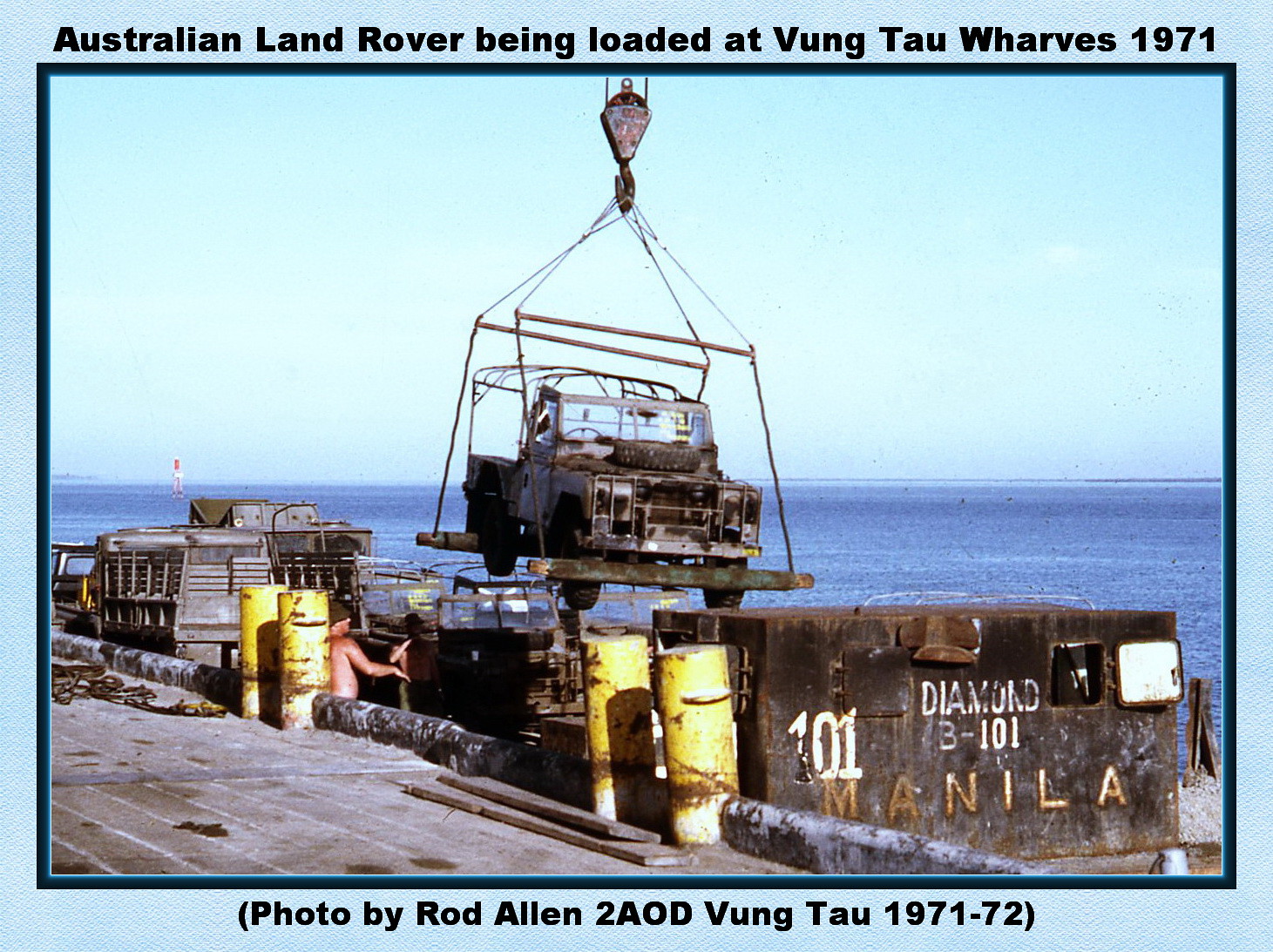In this historical photograph from 1971 at the Vung Tau Wharves, a rusted Land Rover is being carefully lowered by a crane onto a dilapidated boat marked "Diamond 3-101" and "Manila." The setting reveals a bustling port scene against a bright, sunny day with blue skies and water in the background. The boat, positioned adjacent to a dust-covered wooden dock, has yellow posts lining the edge. The Land Rover, hanging approximately five or six feet off the boat’s deck, is guided by a shirtless soldier standing onboard. The visual composition is framed with a light blue border and a darker blue border. Above and below the image, the caption reads: "Australian Land Rover being loaded at Vung Tau Wharves, 1971." At the bottom, a footnote states, "Photo by Rod Allen, 2 AOD Vung Tau, 1971-72." Additional elements include scattered yellow barrels on the dock, indicating ongoing port activities, and another vehicle already stationed on the rusted boat.